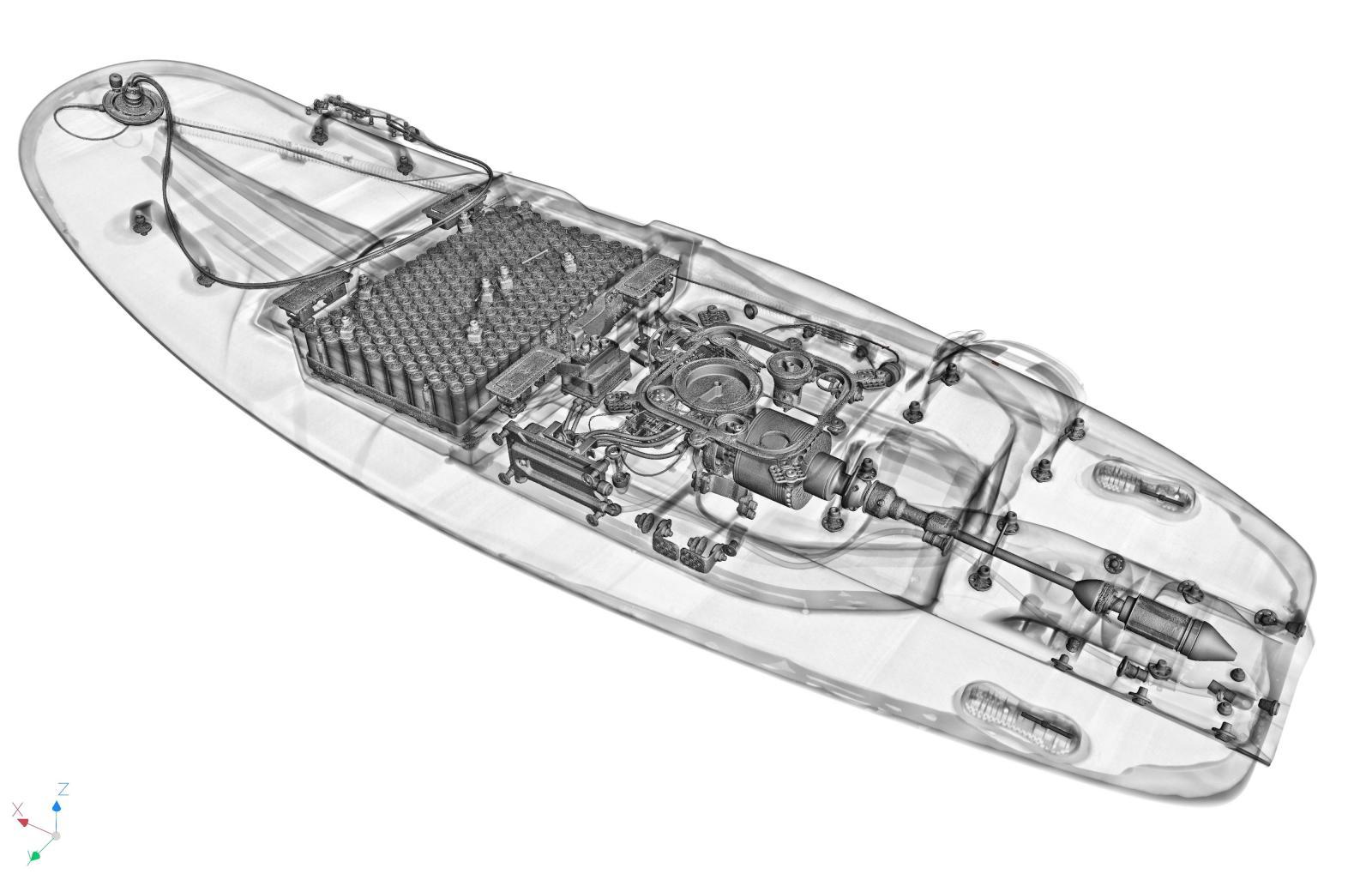The image showcases a grayscale or X-ray-like view of a long, paddleboard-shaped device, revealing its internal components. The see-through board displays an array of cylindrical battery cells clustered towards the forefront, interconnected by various wires. A central motor unit is prominently featured, equipped with belts, wires, and pumps, and a shaft extending towards the back. This shaft suggests the possible attachment of a propeller, indicating that the device is likely a battery-powered electric boat or an advanced paddle board with motorized capabilities. Throughout the board, there are also ropes tied around, adding to its complex internal structure.